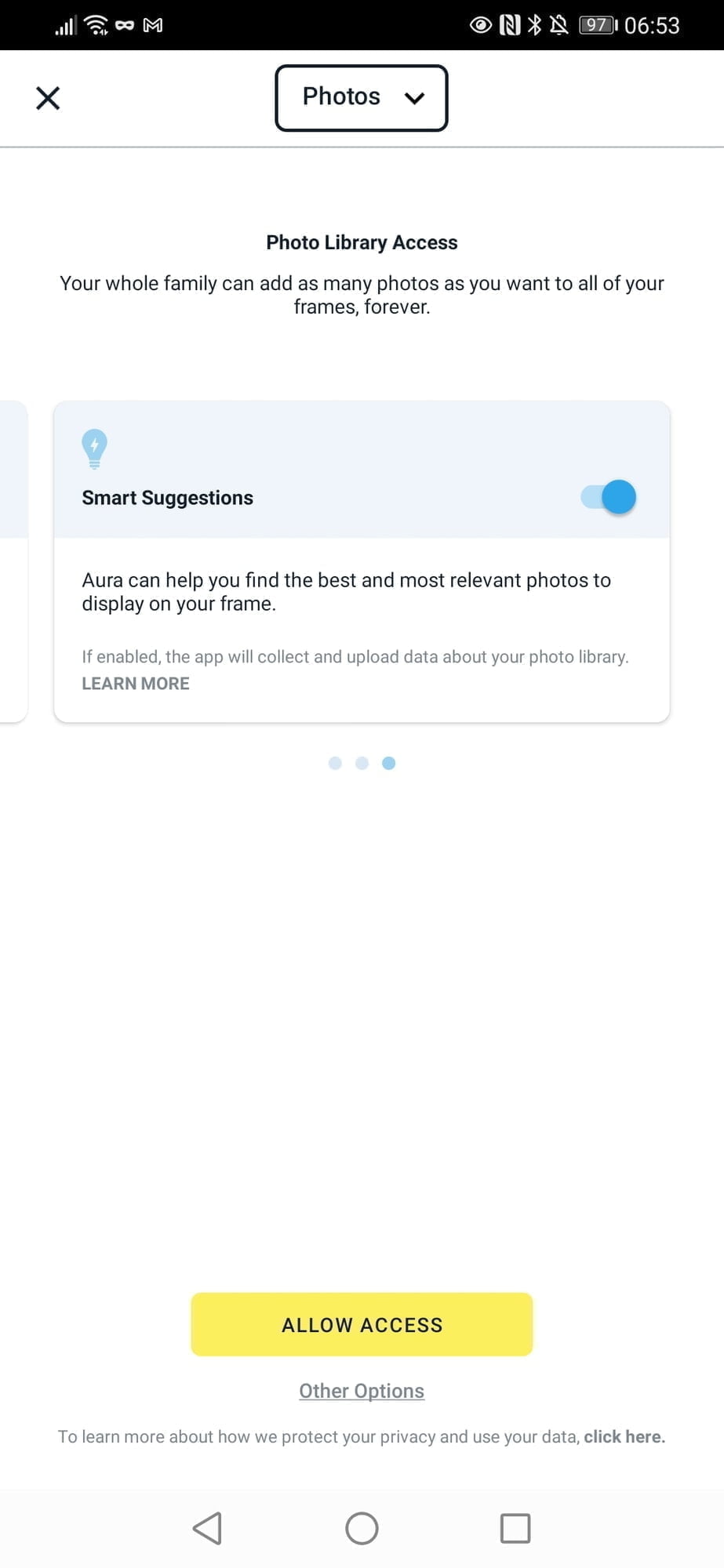This is a detailed screenshot of a mobile application interface. At the very top of the screen, the black notification bar displays several icons on the left including signal strength, Wi-Fi strength, and two additional unidentified icons. On the right side of this bar, the battery indicator shows 97%, and the current time is 6:53. 

Directly below this black bar, on a white background, a header labeled "Photos" is centrally placed near the top. To the left of this, there is an 'X' button. Below the header, text reads, "Photo library access: your whole family can add as many photos as you want to all of your frames forever."

Further down, a section titled "Smart Suggestions" appears within a bordered box. The top half of this box is a very light blue, while the bottom half remains white. The light blue section contains a toggle switch labeled "Smart Suggestions," which is turned on and positioned to the right. The white section describes the feature: "It can help you find the best and most relevant photos to display on your frame. If enabled, the app will collect and upload data from your photo libraries. Learn more."

At the bottom of the screenshot, there is a prominent yellow button with black text that reads "Allow Access." Directly below this button, outside of the bordered box, additional clickable options are displayed. At the very bottom, a smaller gray box contains the text "To learn more about how to protect your privacy and use your data, click here," accompanied by three small icons.

This screenshot captures the various elements and functionalities of the app's photo library access feature, emphasizing the "Smart Suggestions" tool and privacy options available to the user.